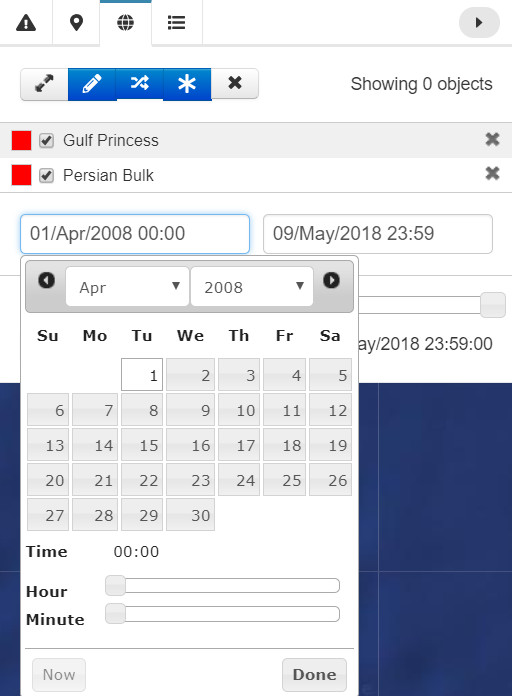Screenshot of a mobile travel site, possibly for booking or tracking cruises. The interface lists two vessels, the Gulf Princess and Persian Bulk, each marked with check marks suggesting selection options. No actual images of the ships are visible. The user can enter travel dates, with an example showing a start date of April 1, 2008, and an end date of May 9, 2018, indicating a ten-year selection span, though this seems unusually long for a cruise. A calendar widget for selecting dates obstructs part of a small map below, revealing only a blue background. The site features various clickable buttons and toggles, though their functions are unclear. The overall context appears to be related to nautical journeys or cruise ship bookings.